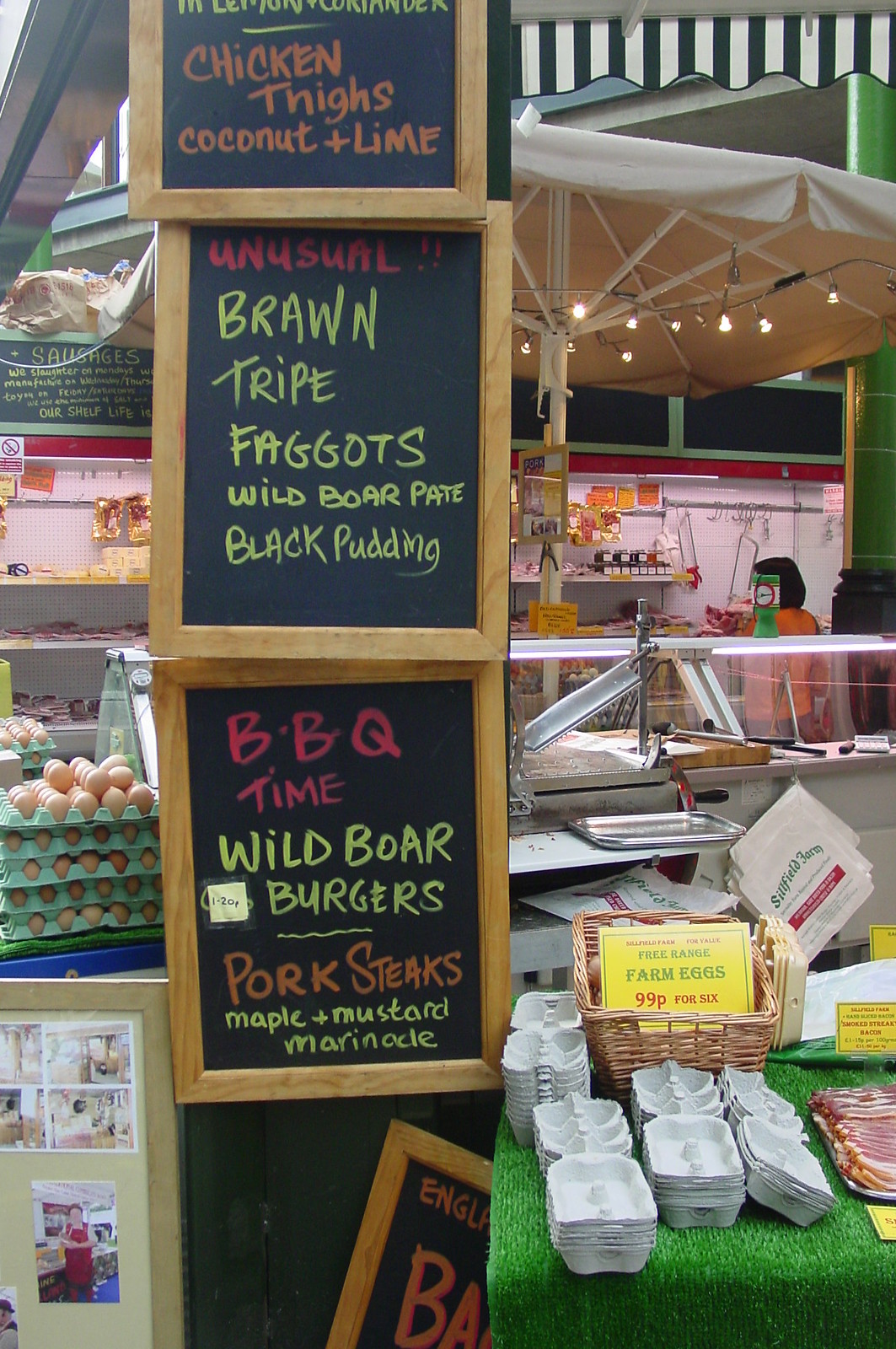In the colorful and bustling scene of an outdoor farmer's market, various foods and festive details converge to create a rich tableau. At the forefront, chalkboard signs with wooden frames display an array of enticing offerings such as chicken thighs with coconut lime, brawn tripe, wild boar, barbecue thyme, wild boar burgers, pork steaks, and sausages, presenting a mix of familiar and exotic meats. These signs are affixed to a green post, which itself stands next to a table covered with green artificial grass, serving as a backdrop for free egg cartons priced at 99 cents each. The table also showcases other breakfast meats, including bacon. A cage laden with crates of fresh eggs adds to the rustic feel, while an umbrella interspersed with lights provides partial shade over some of the food cases. In the background, a refrigerated glass counter suggests the presence of deli or butcher-style offerings, complemented by a white tent overhead and tools hanging on the wall, enhancing the market’s artisanal atmosphere. Just visible off to the side is a woman who appears to be working, contributing to the overall charm and bustling nature of this vibrant, eclectic market scene.